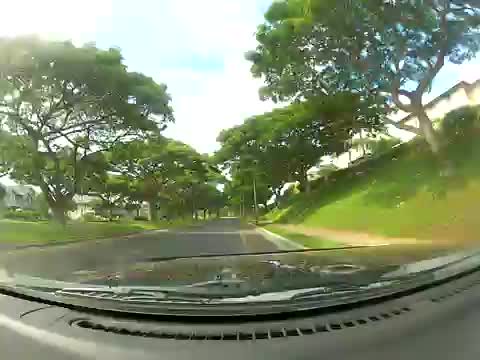An outdoor color photograph, captured through the windshield of a car using a wide-angle or fisheye lens, showcases a slightly distorted but scenic view of a roadway. In the foreground, the car’s dash and black windshield wiper blades are visible, with the dash appearing in gray tones and the hood in dark black paint. The vehicle is moving along a black asphalt road lined with concrete curbs on both sides. 

To the right, a hill rises approximately a story high, covered in lush green grass and dotted with mature, leafy trees. At the base of this hill, a light gray cement walkway runs parallel to the road. On the left side of the road, the terrain is flat but equally rich with green grass and tree-lined, featuring numerous deciduous trees with large canopies extending towards the horizon. 

In the background, distant, indistinct two-story homes are visible on both sides. The sky above is a mix of blue expanses and fluffy white clouds, bathed in good lighting despite the slightly out-of-focus nature of the photograph. There are no text, words, or prints within the image, focusing purely on the scenic drive through this verdant, suburban area.